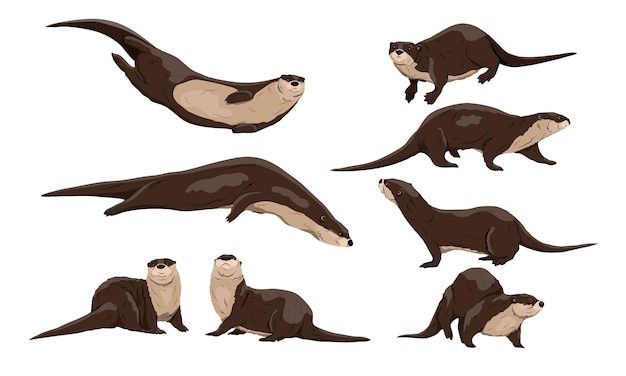The image is a cartoon depiction featuring eight views of a brown and beige sea otter with smooth fur, illustrated against a white background. The top left image shows an otter’s belly from a side angle, swimming off to the right. Directly below this, another otter is belly down, swimming with a hunchback, also moving to the right. At the bottom, two otters are positioned facing each other, one with its face directed to the right and the other to the left, their tails extending in opposite directions. On the top right, an otter faces left with its tail to the right, while below it, an otter is walking to the right on all fours. The next otter down is walking to the left, and beneath that is an otter walking towards the viewer. These simple, yet expressive illustrations capture a variety of poses and orientations of the otters, highlighting their playful nature.